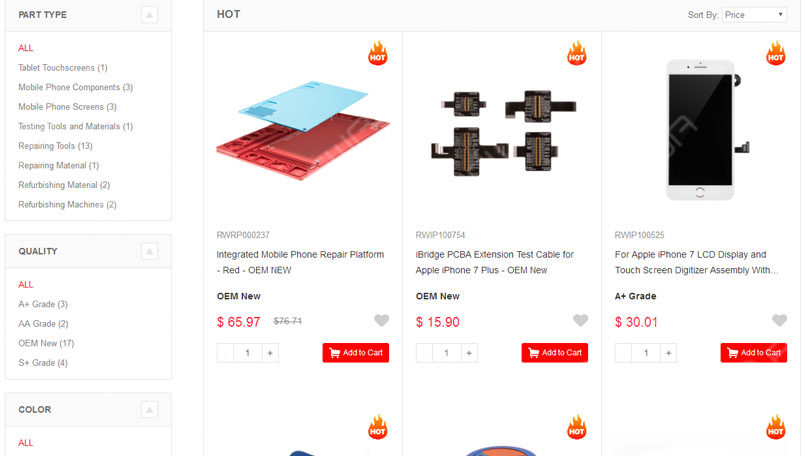Here is a detailed and cleaned-up caption for the image:

---

The image displays a screenshot from an unidentified e-commerce website with a zoom level of 200%. The website features various items available for purchase, each accompanied by an "Add to Cart" button. However, the specific nature or purpose of the website is not immediately clear. On the left-hand side, there is a column of filters—referred to as part type, quality, and color—with all currently set to "all." 

To the right of these filters, several items are showcased, prominently labeled "hot" with a flame icon in the upper right corner of each item, indicating their popularity or special status. Though the main focus is on three completely visible items, there are partial views of three additional items below. 

One notable example among the displayed items is an "integrated mobile phone repair platform." The other items also appear to be related to technology, suggesting the website specializes in tech-related products. 

---

This revised caption provides a clearer and more detailed description, making the context and content of the image easier to understand.